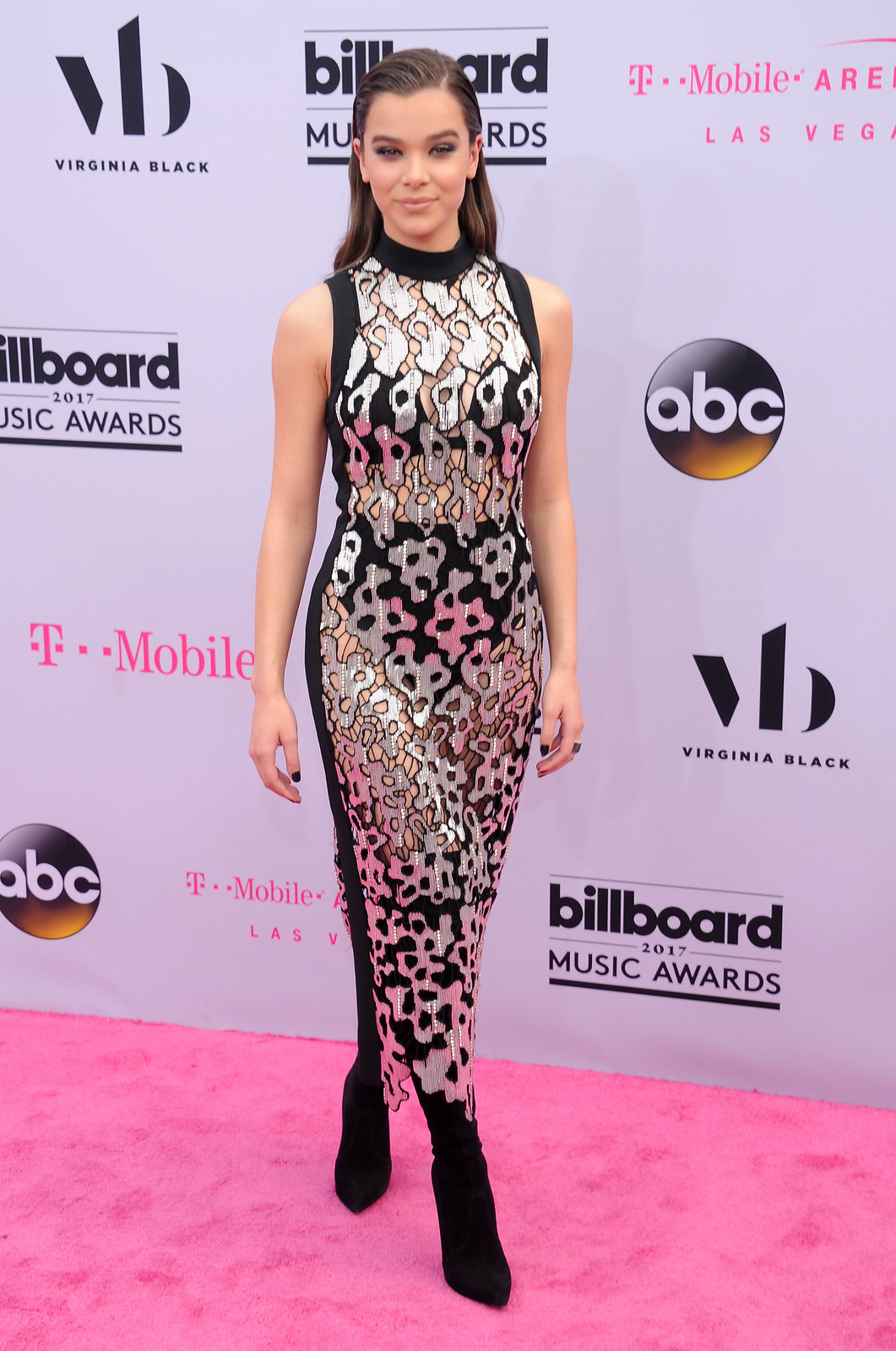The image captures a young woman, possibly an actress or model, posing at what appears to be the Billboard 2017 Music Awards. She is standing on a dark pink carpet in front of a backdrop covered with repeated logos, including ABC, Billboard, T-Mobile, and Virginia Black. Her straight brown hair is pulled back behind her shoulders, and she gazes directly into the camera. She wears a sleeveless, fitted dress with an abstract pattern in silver, gold, and black, featuring sheer cutaways that reveal a black bra and shorts underneath. The dress is complemented by ankle to knee-length black boots with pointed toes and high heels. She also appears to be wearing black nail polish and a ring.